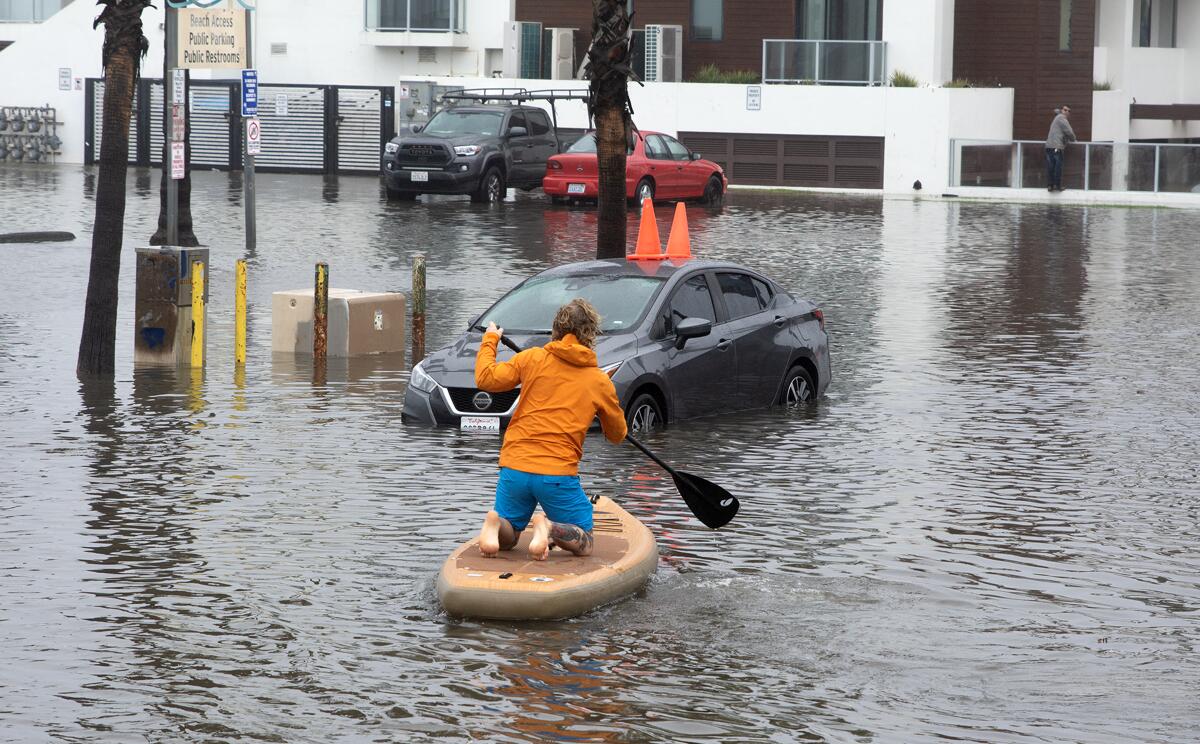In a city street overwhelmed by floodwaters, a person in an orange raincoat with a hood, blue shorts, brown high boots, and a tattoo on their right leg kneels on a brown paddleboard and uses a black paddle to navigate past several partially submerged cars. The flooded car in the center is a dark gray Nissan, its windows up and too inundated to be driven, with two cones placed on its roof. The surrounding scene features large brown-and-white apartment buildings with fencing on top, a partially visible pine tree, and a sign in the top left corner indicating "Beach Access, Public Parking, Public Restrooms." Amidst the rainfall, another person in a gray jacket and jeans stands on a nearby ledge, holding onto a building's edge to keep out of the water.